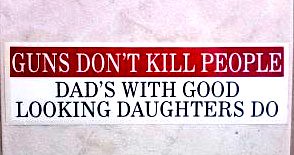The image depicts a rectangular sign in a landscape orientation, positioned centrally on a pink marble background with light gray veins. The sign has a white background with a red banner at the top. The red banner features white text in large capital letters stating, "GUNS DON'T KILL PEOPLE." Below this, centered on the white background, is black text also in large capital letters that reads, "DADS WITH GOOD-LOOKING DAUGHTERS DO." The sign covers the width of the photograph, extending from the left to the right side, with some space above and below it. The photograph is taken in a realistic, representational style, emphasizing the humorous nature of the sign, which might resemble a bumper sticker.